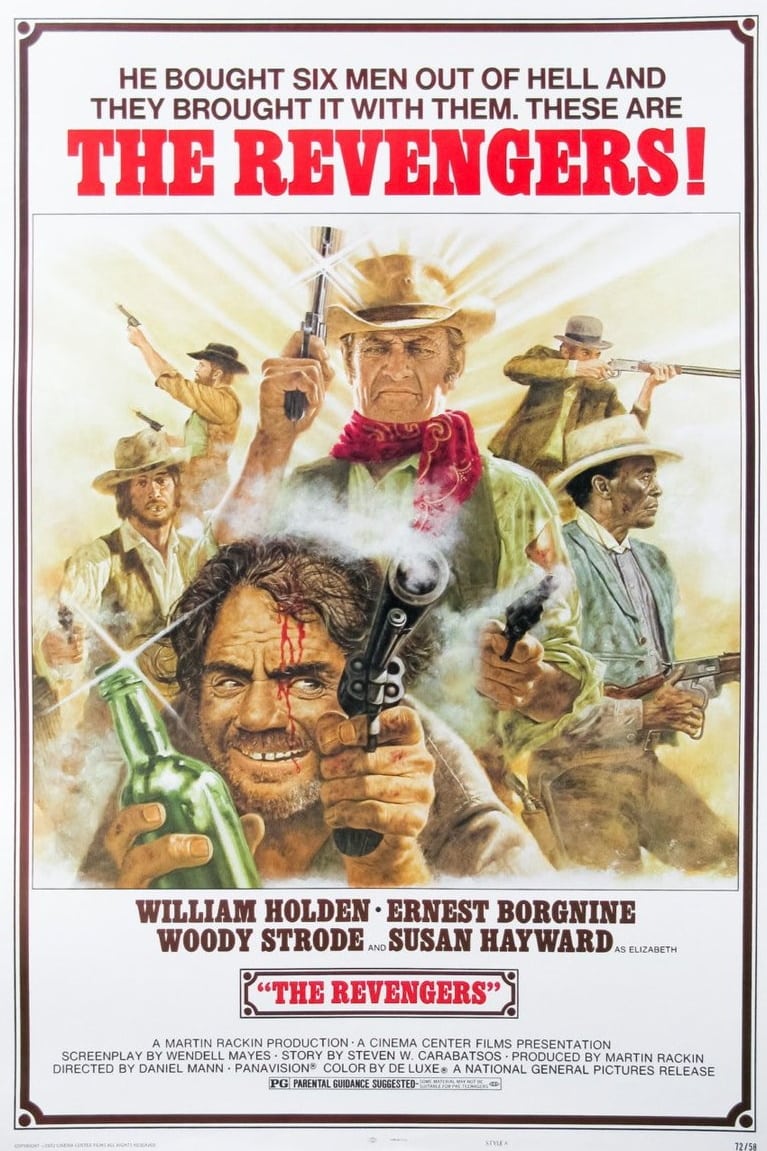This detailed movie poster for a western-style film, titled "The Revengers," features an eye-catching collage of six rugged cowboys. The central figure, a cowboy with a revolver in each hand and a red handkerchief around his neck, stands out prominently. In the foreground, another cowboy, blood streaming down his face, points a revolver at the viewer while holding a green glass bottle. Flanking the central figures are two cowboys on the right, each in brimmed cowboy hats and clutching lever-action rifles, and two more on the left, each brandishing pistols in both hands. All the characters wear traditional cowboy hats, contributing to the classic Western aesthetic.

The text at the top of the poster reads, "He brought six men out of hell and they brought it with them. These are The Revengers," with "The Revengers" emphasized in large, bold red letters. Below the illustration, the stars of the film are listed: William Holden, Ernest Borgnine, Woody Strode, and Susan Hayward as Elizabeth. The poster also includes production credits, noting it as a Martin Rackin production, a Cinema Center Films presentation, with a screenplay by Wendell Mays and a story by Stephen W. Carabazos. The film is produced by Martin Rackin and directed by Daniel Mann, shot in Panavision and color by Deluxe, and is released by National General Pictures with a PG rating.